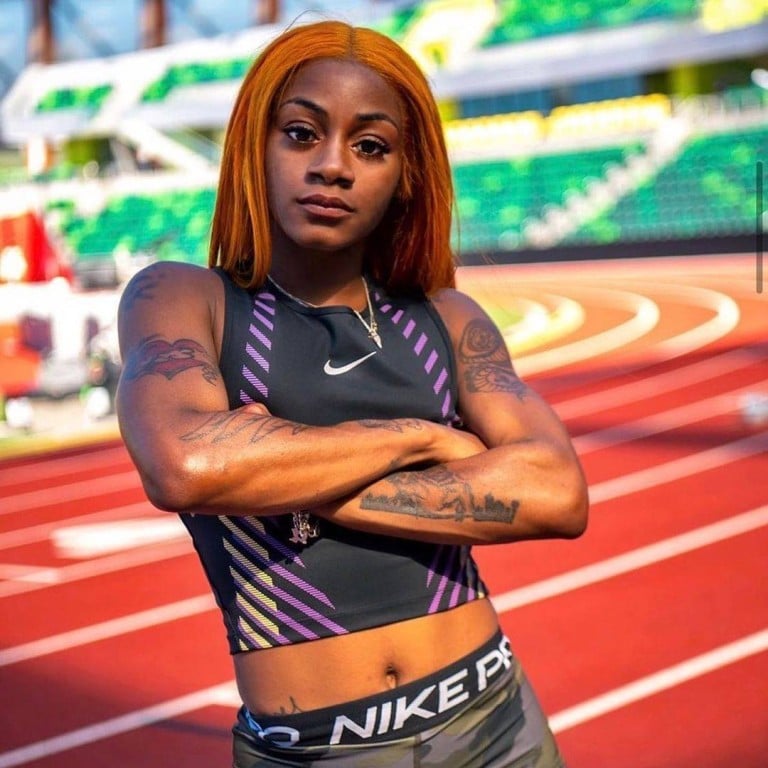This large square image showcases a close-up shot of a serious-looking female athlete, likely a runner, standing on a track field with a set of green bleachers and white steps visible in the background. She appears to be of African-American descent, with striking orangish-red hair parted in the middle and straight, cascading down. Her dark skin contrasts beautifully with her attire, as she stands confidently with her arms crossed over her chest, displaying her numerous tattoos across her biceps and forearms. She wears a black Nike crop top adorned with white and purple stripes, and Nike Pro shorts that feature a purple, black, and camouflage pattern. The shorts prominently display the Nike logo on the waistband. The athlete's large brown eyes and stern expression enhance her tough and focused demeanor, making her a striking and powerful presence in the image. The sunny weather illuminates the scene, highlighting the details of both the runner and the track field around her, with its distinct yellow, red, and white lane markings.